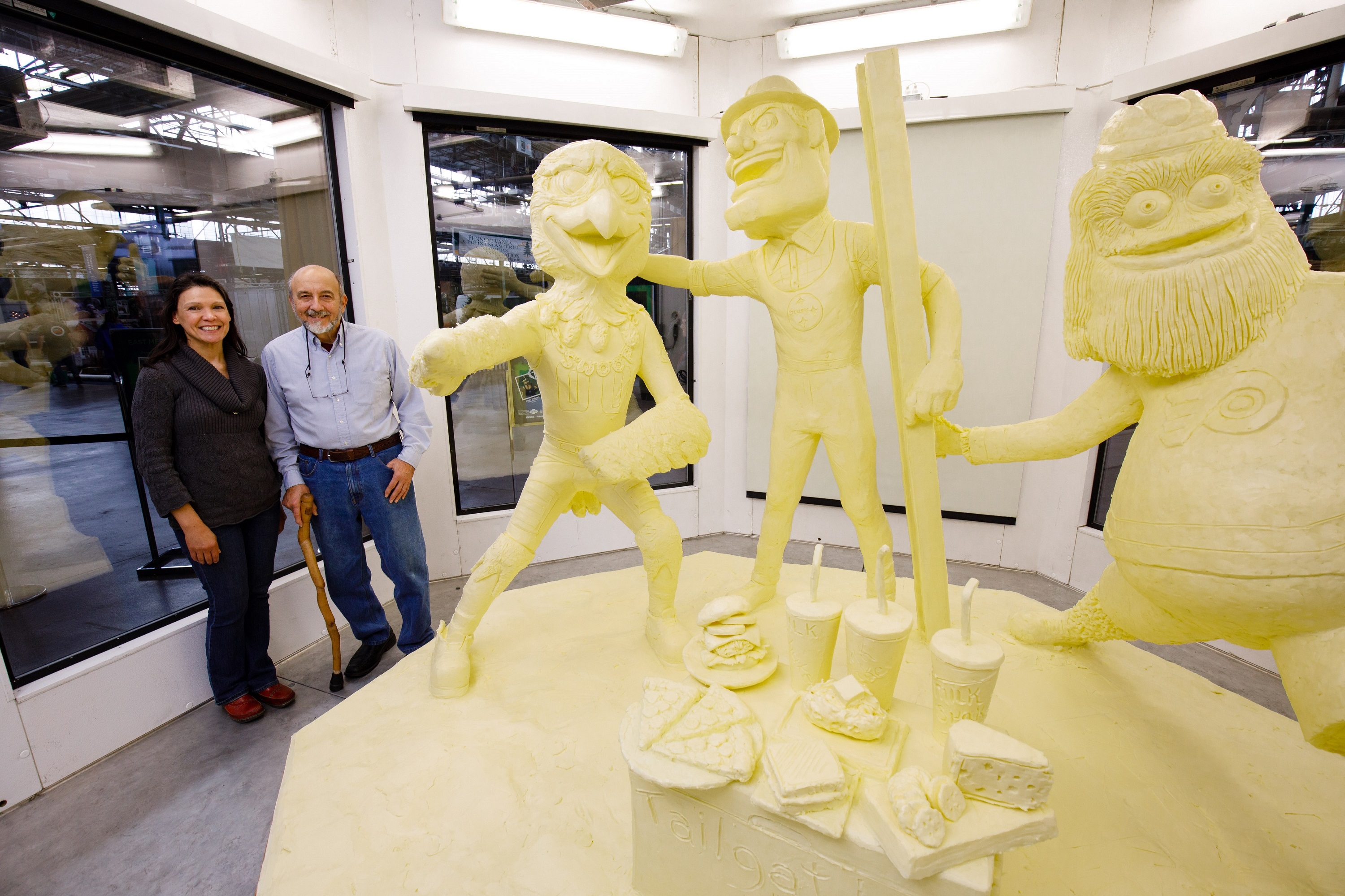The photograph captures a brightly-lit indoor room shaped like an octagon, where nearly each side is composed of large windows that flood the space with natural light. The interior walls are painted white, with one window partially covered by blinds. In the center of the room sits a pedestal displaying intricate sculptures resembling three animated figures, each carved with distinct features. One figure is depicted with a beak, another with a pronounced ear, and a third, rotund. These sculptures, colored a creamy yellow akin to butter, are surrounded by carvings of various foods, including cheeses and crackers.

Two people stand near the left side window, their reflections visible against the glass. The woman, who appears to be middle-aged, has long dark hair, a medium skin tone, and is dressed in a sweater, jeans, and red shoes. The older man beside her sports a blue shirt, blue jeans, a small beard, and uses a cane with his right hand for support. The detailed depiction of the scene portrays a harmonious blend of natural light, human presence, and captivating art.